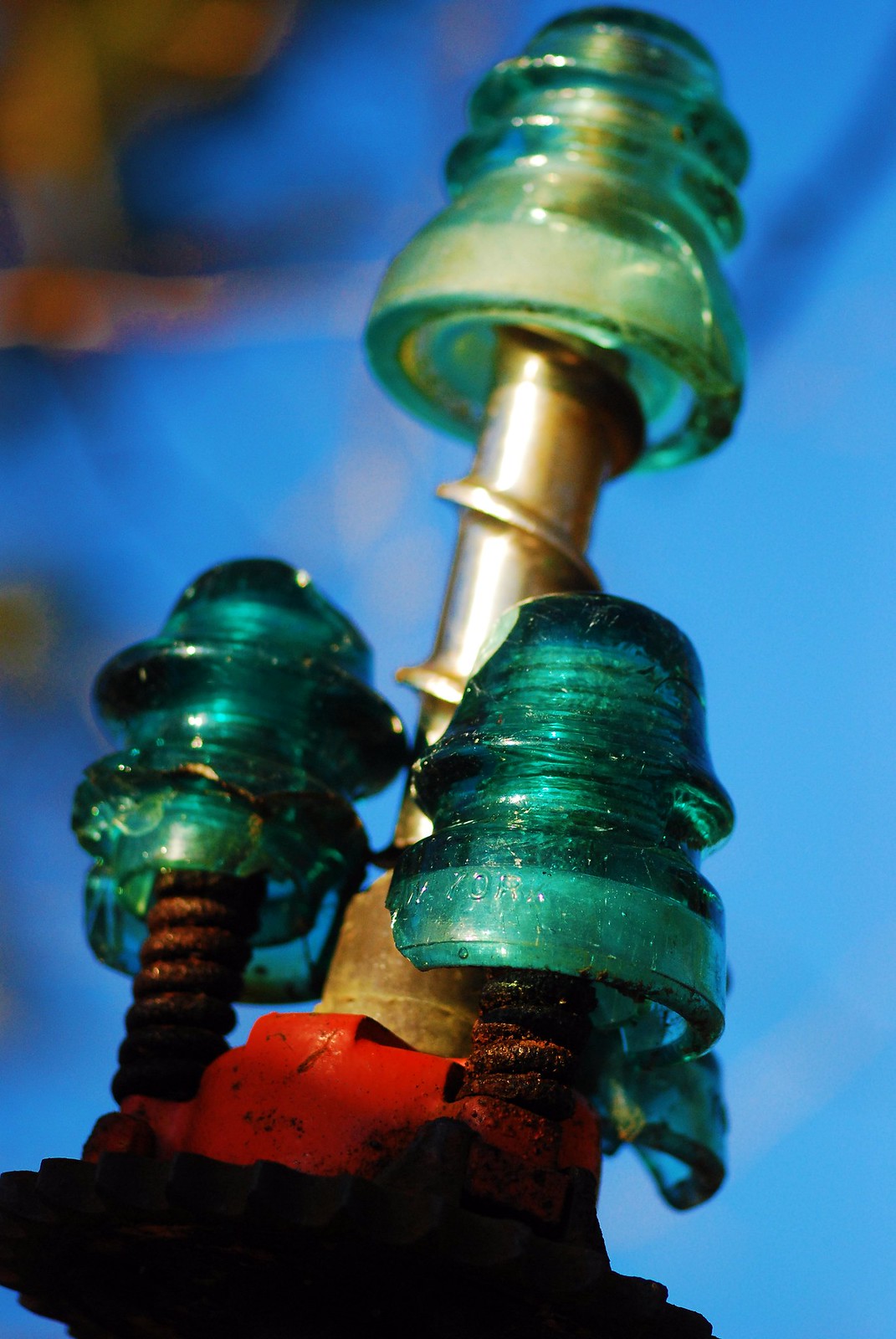This image showcases a detailed close-up of intricate equipment that includes three transparent, green glass rods or handles attached to the ends of metal coils or rods, suggestive of transformer components. These green components, which might appear as clear ear pieces, are affixed to both regular and wood-like screws. The scene includes a predominantly blue-colored background with a blurry effect, enhanced by an orange reflection in the upper left corner and a prominent red metal base that appears rusted. The entire setup is illuminated, highlighting the transparency and details of these glass rods, with one of the rods appearing lighter in color than the others.